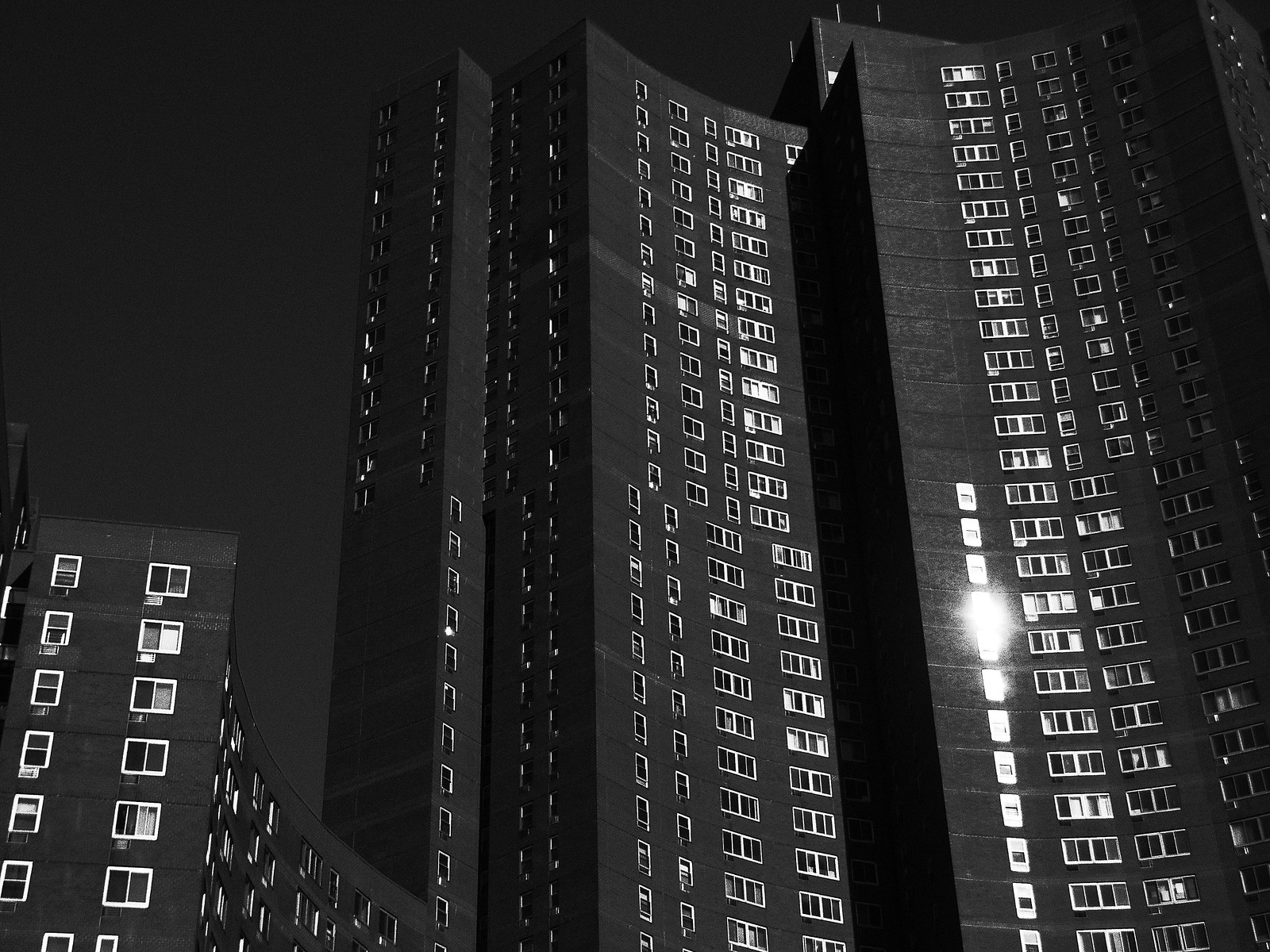The image, likely a digitally created cityscape, depicts a stark, dystopian scene dominated by several skyscrapers aligned in a semicircular pattern. Each building features a distinctive concave curve and rises to an imposing height of 20 to 30 stories. The structures are primarily black, accented only by silver trim around the windows, contributing to a streamlined, monolithic appearance. The sky in the background is an impenetrable black, enhancing the dark, futuristic ambiance. To the left, a shorter building, approximately 10 stories tall, curves into the near foreground, diverging slightly from the more uniformly tall towers. This shorter structure, like its taller counterparts, is also entirely black with silver window trim. The buildings have numerous rows of windows, some of which seem to open and may even contain air conditioning units, suggesting a residential or multi-use function. The overall image is in black and white, with the dark sky and silver reflections on the windows indicating it may be captured at night or presented in a monochromatic palette. Despite the absence of celestial bodies, the sunlight or another light source reflects off some windows, adding subtle highlights to the otherwise dark cityscape.